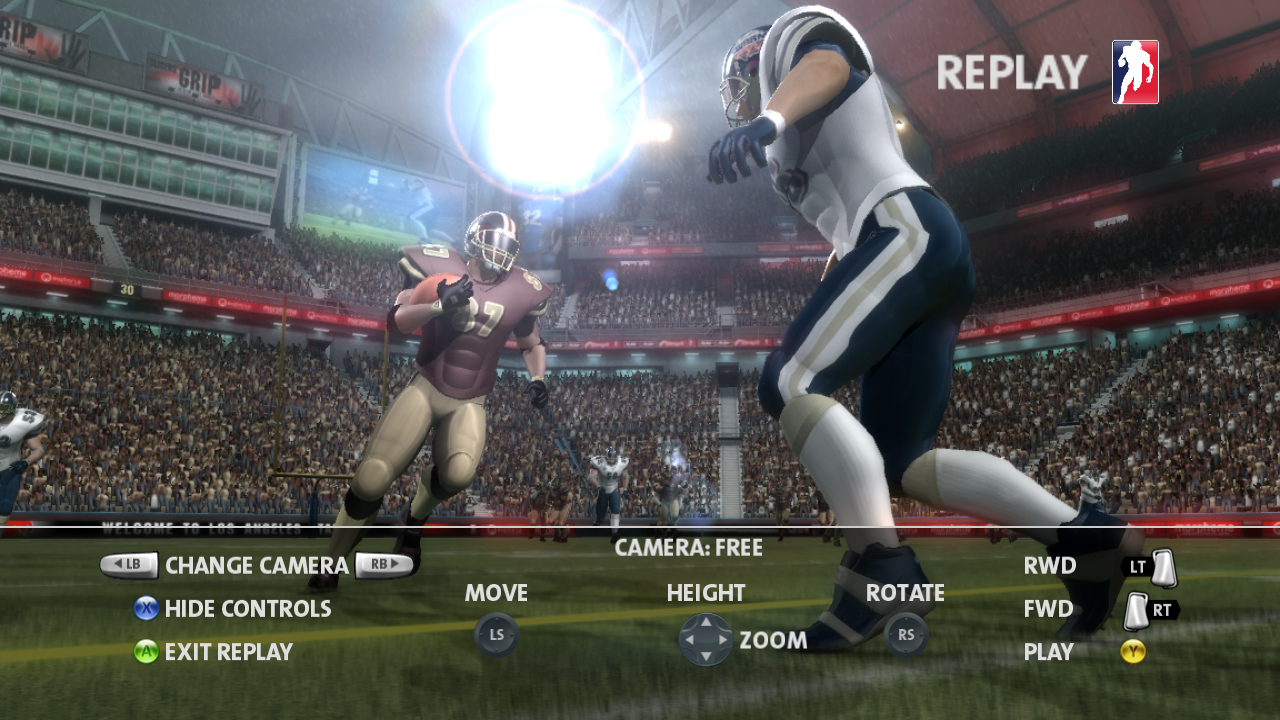A detailed gameplay capture of an NFL video game, showcasing an intense moment on the field. One player, sporting a uniform of white, navy, and gold, stands poised against an opponent clad in burgundy, gold, and black. The lush, green field is marked with crisp yellow and white lines, clearly indicating yardage and boundaries. Surrounding the field, the stadium is packed with what appear as brownish blobs symbolizing the cheering crowd. Above the stands, red and white digital scrolls provide updates and information. Illuminating the scene, an overhead light ensures the action is well-lit. In this particular snapshot, the player in burgundy and gold is tightly gripping the football, ready to make a decisive play. At the bottom of the image, a user interface overlaid with various icons in gray, blue, green, white, and gold provides options such as "change camera," "hide controls," "exit replay," "move," "camera free," "hide," "zoom," "rotate," "fast forward," "rewind," and "play" for an enhanced viewer experience.